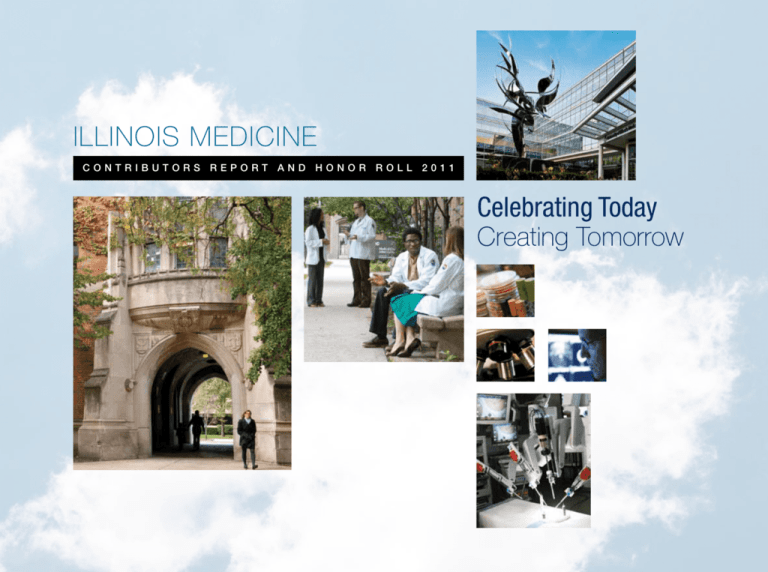Front cover of the digital magazine "Illinois Medicine," featuring a serene blue sky with scattered clouds as the background. The title "Illinois Medicine" is prominently displayed at the top. Directly below the title is a black banner with white text that reads, "Contributors Report and Honor Roll 2011." 

On the right side, there's a small insert image showing the university campus, highlighting a notable metal art installation on the quad and showcasing the campus's modern architectural design with expansive glass panels. Beneath this image is a slogan that reads, "Celebrating Today, Creating Tomorrow."

Below the banner and slogan, there are four smaller images, each depicting different aspects of the medical field. One image is a close-up of a microscope, another showcases a research laboratory, while another provides a view of a building entrance with an arched walkway, bustling with people entering and exiting. The final image portrays a campus walkway lined with benches, where medical school professionals are seen engaging in conversation.